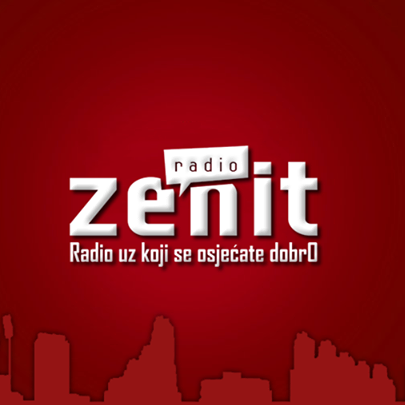The image is a detailed advertisement for the radio station "Radio Zenit." The prominent feature in the middle is the name "ZENIT," written in lowercase, white embossed letters. Directly above "ZENIT," there is a smaller rectangular speech bubble with the word "Radio" in red letters on a white background, creating a dialog box effect emerging from the letter E. Below "ZENIT," a foreign language sentence starting with "Radio uz kojo cse osjecate d obr" is displayed in white text. The background features a gradient from a deep blood red around the edges to a lighter red in the center, highlighting the central text. At the bottom of the image, there is a subtle outline of city buildings, likely European, represented in a lighter red hue that blends with the background. Overall, the poster uses a simple yet striking red and white color scheme to draw attention to the name and details of the radio station.